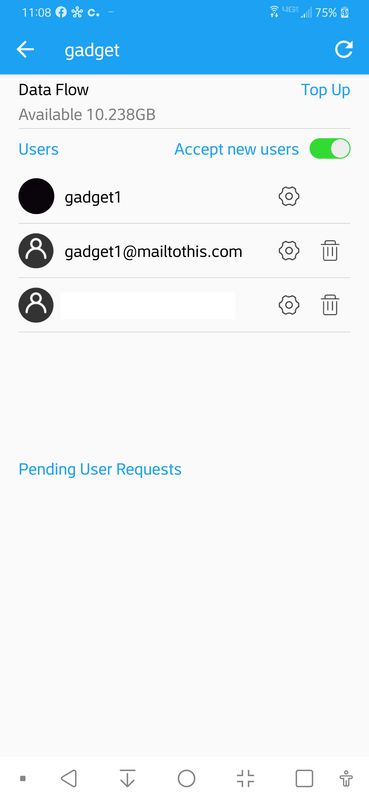This image is a detailed screenshot from a cell phone display. 

At the very top, approximately one-eighth of the screen is occupied by a blue taskbar. On the left-hand side of this taskbar, in white text, the time reads "11:08." Next to this, the white Facebook logo is visible, followed by what appears to be a snowflake icon and a 'C' with a period. To the far right of the taskbar, there are several icons indicating the phone's status: the Wi-Fi symbol with active up and down arrows, a 4G LTE icon, a signal strength indicator showing about two out of five bars, and a battery icon indicating approximately 75% charge.

Just below the taskbar, on the left side of the screen, there is a white back arrow beside the white word "gadget" and a white half-circle with an arrow. Below this area, the background transitions to a gray or white hue.

Starting at the top left of this section, "Dataflow" is written in black text. Underneath it, "Available 10.238 GB" is displayed. To the right of this text, the word "Top up" is highlighted in blue. Beneath this heading is a blue line labeled "Users" followed by a toggle option to "Accept new users," featuring a green on/off switch with a white dot.

Further down, there are three black squares lined up vertically. The top square, labeled "Gadget one," features a settings icon beside it. The middle square reads "Gadget one at melvis.com" and includes both settings and trash icons. The third square is a blank white box, also accompanied by settings and trash icons. 

Below these squares is the blue text "Pending user request."

At the very bottom of the screenshot, there is a horizontal white bar with several control icons. These include a dot, a backward play button, a download button, a circle, a full-screen toggle, a white square, and a small person icon.